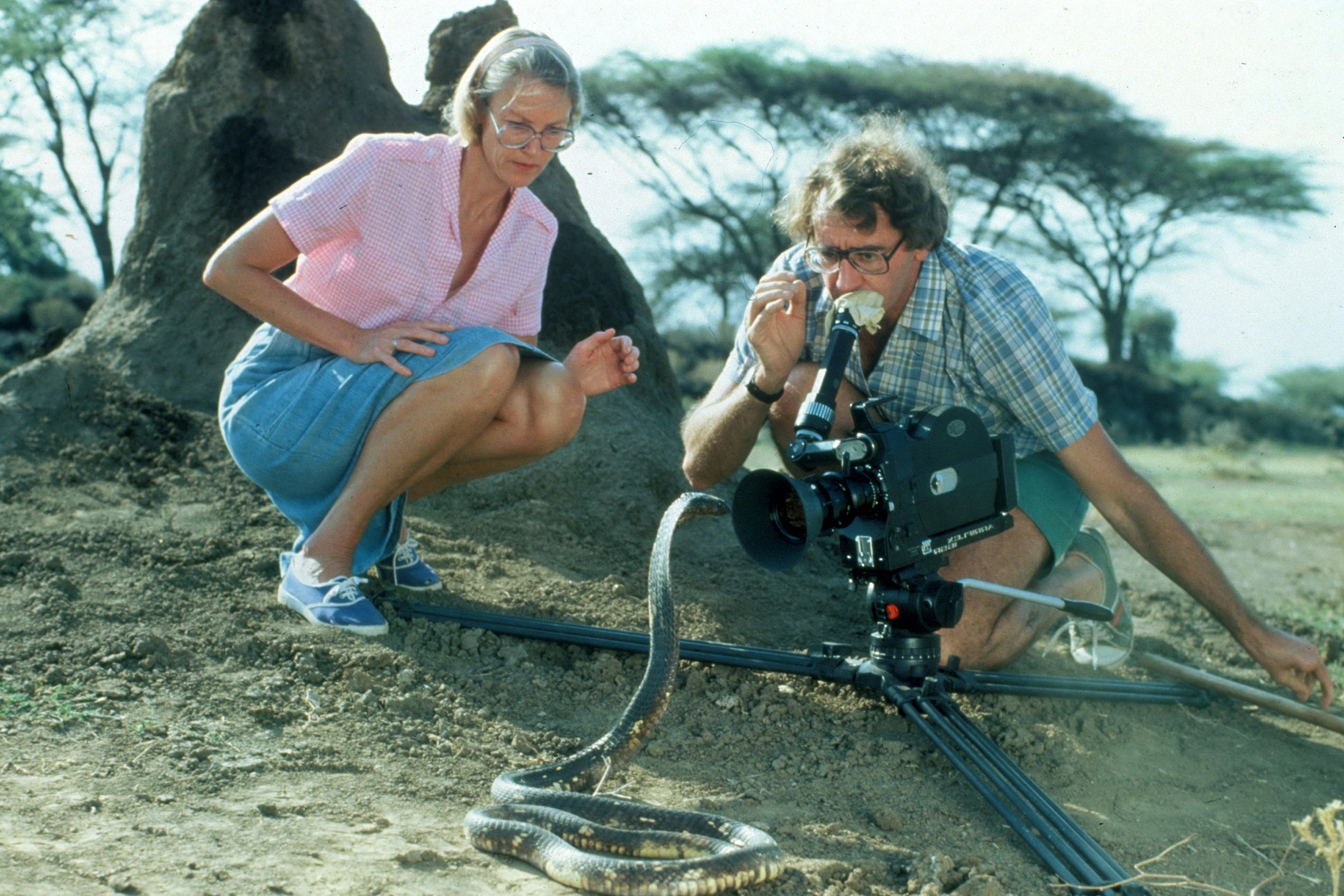In this outdoor photograph set in a natural environment with blurry trees in the background, an older woman and a middle-aged man are captured kneeling on light brown dirt ground, closely examining a snake, likely a cobra, with its head raised in an alert posture. The woman, who appears to be in her 50s or 60s, has gray hair and is dressed in a pink shirt paired with a blue denim skirt and shoes. Beside her, the man, appearing to be in his 40s or 50s with gray curly hair, wears a black and white striped shirt, blue shorts, and gray shoes. They are equipped with a serious, old-school film camera mounted on a low tripod, aimed directly at the cobra for a close-up shot. The man is carefully positioning the camera, while the woman, squatting nearby, observes the snake intently.